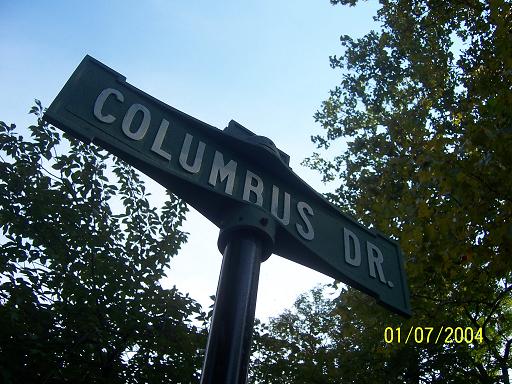In this vibrant outdoor photograph, we observe a lovely scene framed by a clear blue sky adorned with a solitary, powdery white cloud stretching across the lower portion. Central to the image is a hunter green street sign, viewed from a perspective as if standing directly beneath it, angled upwards. The sign prominently displays the words "Columbus Drive" in crisp white lettering against its green background. Adding a natural touch to the composition, dense tree branches laden with small, pear-shaped green leaves encroach from the left, right, and upper right corners, offering a lush contrast to the clear sky and structured street sign. Notably, the lower right corner of the photograph bears a time stamp in yellow text, indicating the date of capture as "01-07-2004."